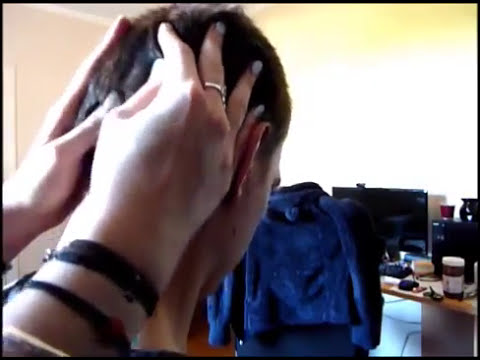In this indoor setting, likely someone's home, a young man with very short black hair is seen from the back as a woman methodically inspects his head, possibly checking for lice. Her hands, adorned with a silver ring on her ring finger and light purple painted nails, are gently pulling through his hair. The young man leans slightly forward, centering the scene around his head and the woman's hands. To the right, a cluttered desk is visible, topped with a monitor, various bottles, papers, and food items. A chair draped with a blue sweater sits in front of the desk. The background features an unadorned yellow wall. The overall image quality is low, with soft details and visible compression artifacts, casting a slightly grainy texture over the scene. The colors present in the image include tan, black, white, blue, yellow, and brown.